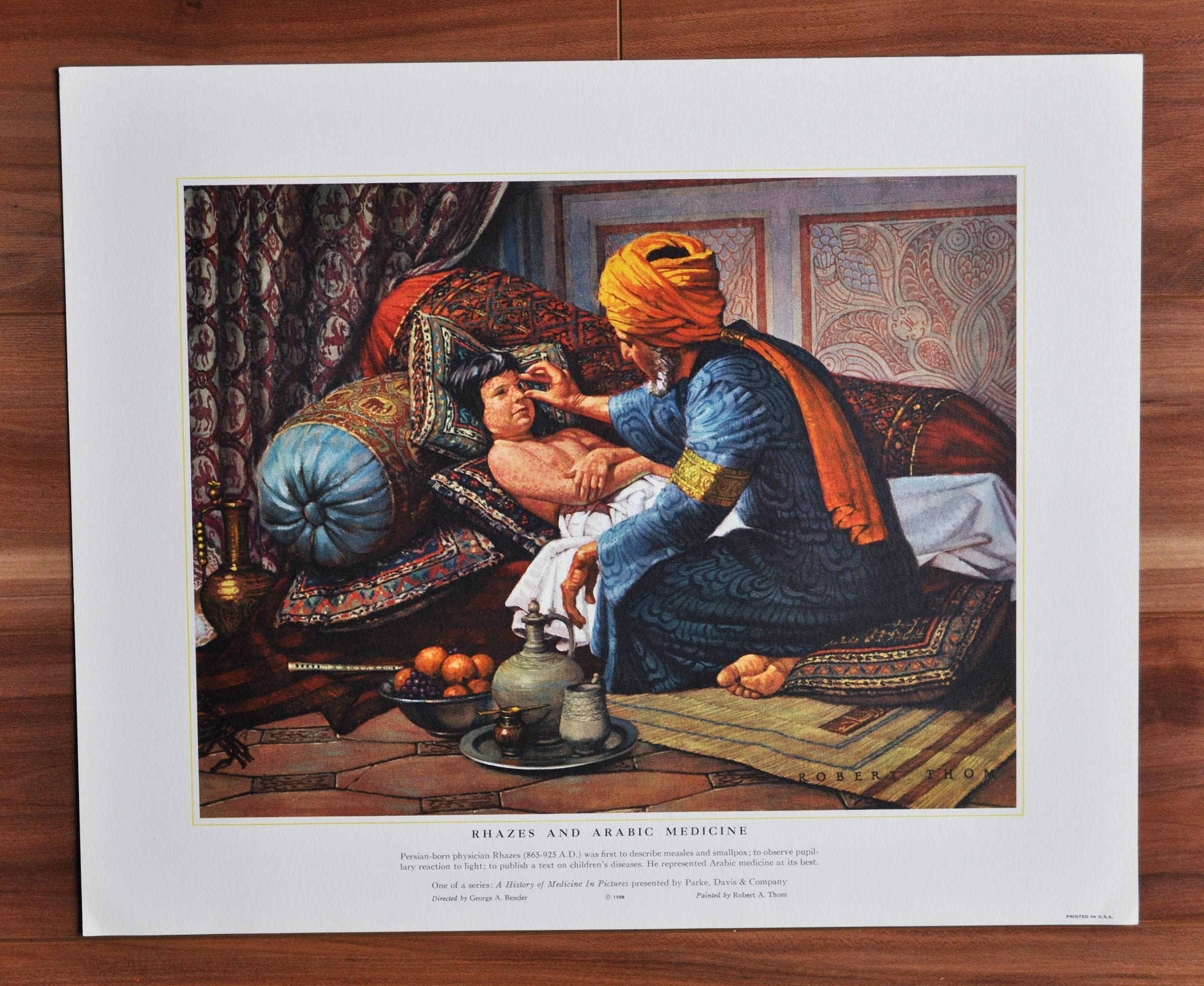The image is a detailed, colorful illustration of a Persian-born physician, Razes, from the series "A History of Medicine in Pictures" presented by Park Davis and Company. The photograph shows the picture resting on a wooden surface, surrounded by a white mat with black lettering at the bottom that spells "RAZES and Arabic Medicine," though some additional text is too small to read clearly. The scene depicted is of a man in a blue robe with an orange turban, sitting cross-legged on a cushion, tending to a child or small person who is shirtless with dark hair, lying on a makeshift bed of patterned pillows and a rug on a tile floor. The man, identified as Razes, is holding the child's eye open, possibly examining it. Surrounding them are various objects, including a bowl of fruit, a ewer of tea with a cup, and a pot, emphasizing the Arabic and Moroccan theme with their intricate designs and bright colors. The backdrop features rich tapestries and possibly a curtain, adding to the ornate setting of an Arabic Muslim home.